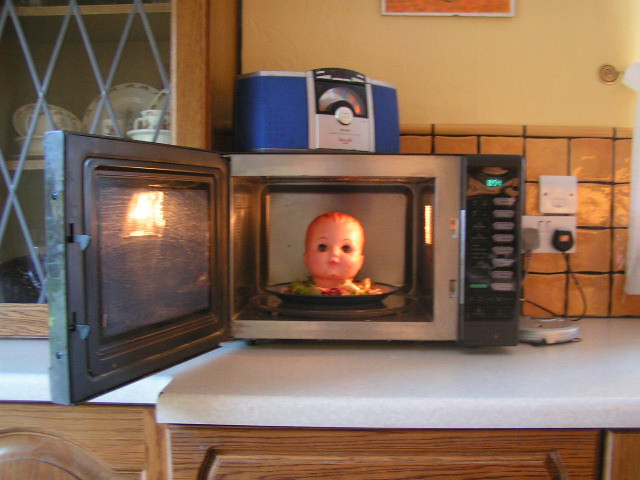This detailed color photograph captures a kitchen scene centering around an open microwave oven positioned on a white marble countertop. The grey microwave, its light on and door fully open, reveals a dark-colored plate, possibly black or blue, bearing a peculiar display: a plastic baby doll's head with short, brownish-orange hair, encircled by various vegetables and what appear to be shreds of lettuce and tomatoes, lending an unsettling, messy impression.

Above the microwave sits a blue and grey boom box, and plugged into a nearby power outlet is a small grey object adding to the scene's eclectic nature. The background features a half-tiled wall of orangey-brown tiles transitioning to a pale beige painted upper section. Adjacent to the microwave is a leaded glass cabinet, showcasing fancy old china with decorative edging visible through its intersecting glass pattern.

This kitchen setup is further complemented by white countertops and brownish wood cabinetry with patterned embossments, creating a contrast in the overall decor. A light fixture on the right and a window with brownish curtains and a greyish frame on the left frame the bizarre focal point—an unexpected blend of domesticity and surrealism.